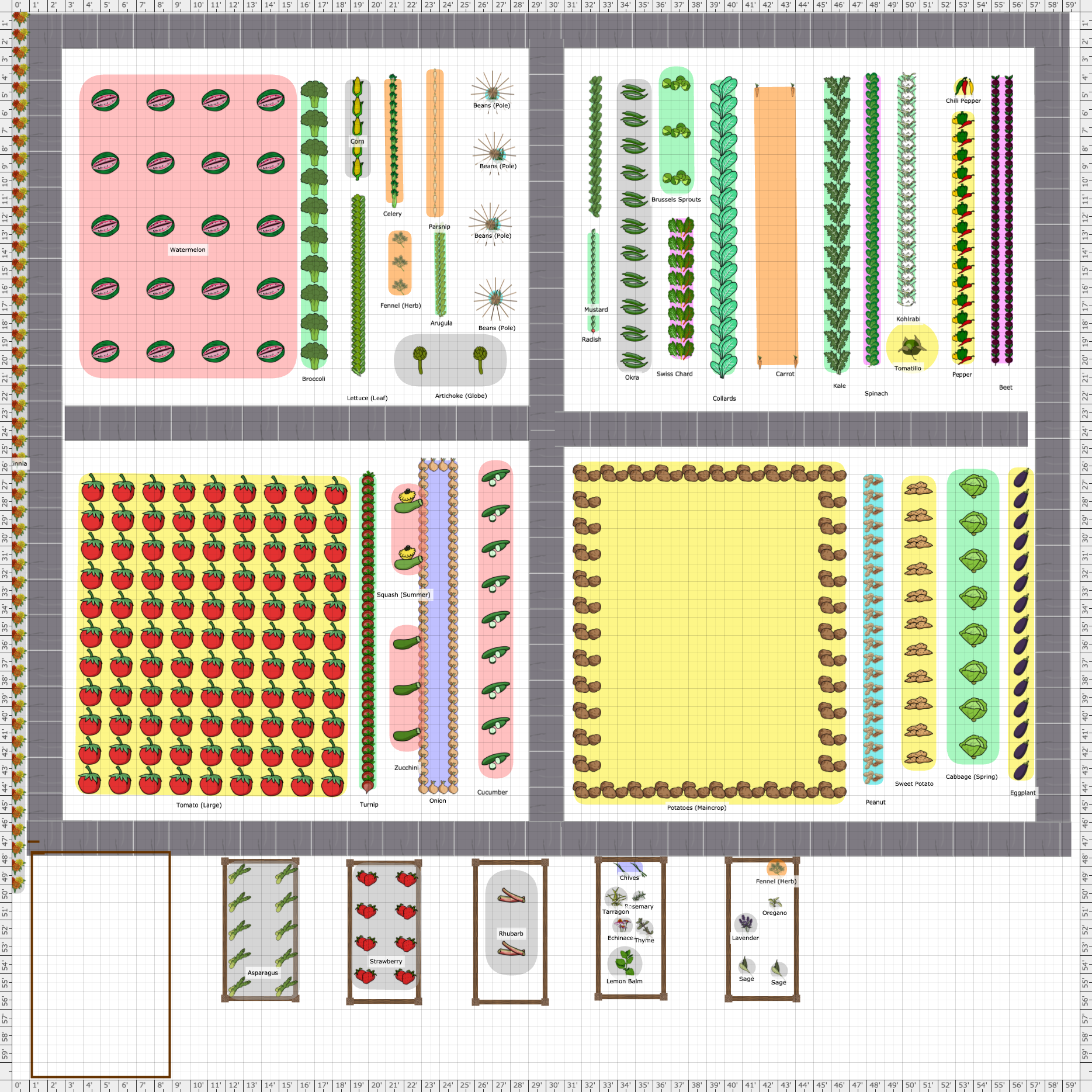The image is a meticulously organized garden plan, laid out on a detailed grid measuring 60 by 60 feet. Each section of the grid is marked by feet on all four sides and features an array of vegetables and fruits planned for cultivation. The top half of the grid is divided into sections with designated spaces for different plants. The upper left area lists varieties such as watermelon, followed by a thin section designated for broccoli, corn, lettuce, celery, and parsnip. The right side of the upper half features a box with a white background, earmarked for growing radish, okra, collards, carrots, kale, peppers, and beets.

On the lower left of the grid, a large area is allotted for tomatoes, adjacent to a smaller section set aside for zucchinis. The lower right features an expansive section for potatoes, flanked by thinner sections designated for peanuts, sweet potatoes, cabbage, and eggplants. Supplemental details include rows and columns interspersed with gray boxes, possibly to aid in the identification and organization process. Accompanying text lists additional plants such as mustard, Swiss chard, Brussels sprouts, spinach, turnips, onions, and cucumbers, all meticulously planned to maximize the garden's productivity and organization.

Overall, this detailed plan serves as a comprehensive guide for planting and managing a diverse garden, ensuring each type of plant has its own allocated space within the grid system.